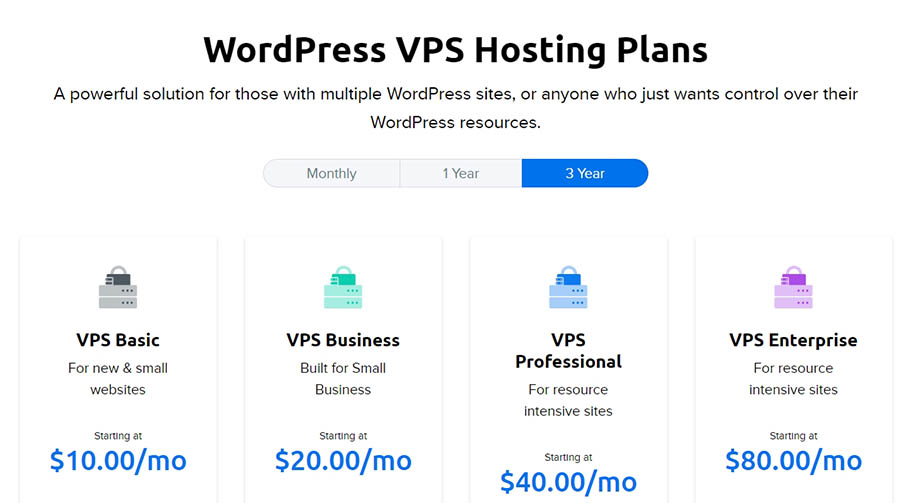Screenshot of WordPress VPS Hosting Plans pricing page. The page headline reads "WordPress VPS Hosting Plans: A powerful solution for those with multiple WordPress sites or anyone who just wants control over their WordPress resources." The displayed options include monthly, one-year, and three-year plans, with the three-year plans highlighted in blue. 

- **VPS Basic**: Ideal for new and small businesses, priced at $10 per month.
- **VPS Business**: Suitable for small businesses, priced at $20 per month.
- **VPS Professional**: Designed for resource-intensive sites, priced at $40 per month.
- **VPS Enterprise**: Also for resource-intensive sites, starting at $80 per month.

Each plan is represented by an icon depicting two server units stacked with a handle, resembling a sideways toaster. The icons are colored differently: gray, green, blue, and purple, respectively. The page has a clean and simple design with a white background, black and light gray text, and prices highlighted in blue font for easy readability.